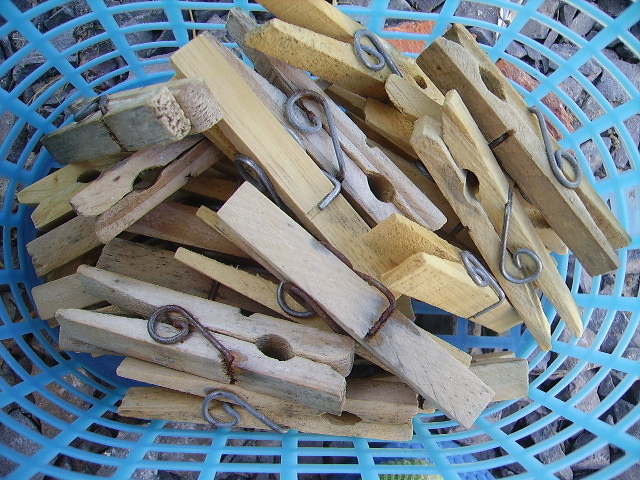The photograph captures a light blue plastic laundry basket, approximately halfway full with old-fashioned wooden clothes pins. These wooden clips, used for hanging clothes to dry, feature metal springs, some of which have developed rust over time, indicating their age. The basket is positioned in an outdoor setting, resting on a surface that appears to be a light brown towel atop a mix of bricks and light gray stones. The basket has openings on all sides, allowing glimpses of the rugged outdoor ground beneath. The photo, taken in bright daylight, focuses closely on the weathered, brown clothes pins, emphasizing their vintage character and the rustic quality of the scene.